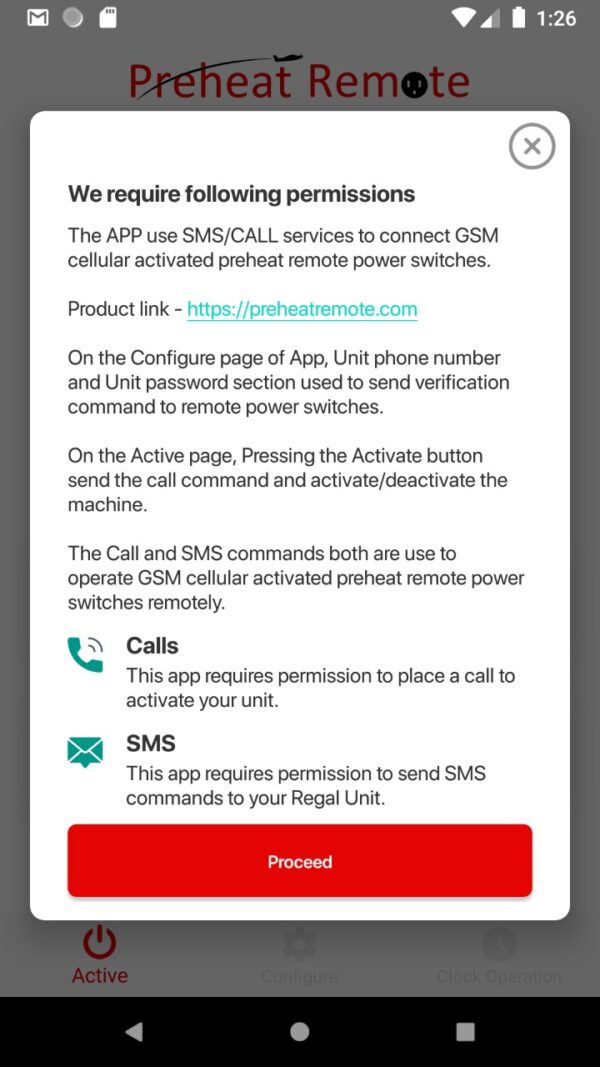In the upper right corner of the image, the battery icon is almost completely full and displayed in white, with the time showing as 1:26. In the background, a dark gray overlay includes the text "Preheat Remote" in red letters. 

Central to the image is a long vertical box containing a detailed permissions request. In black text, it states, "We require the following permissions:". The app notification specifies the use of "SMS" and "CALL" (both capitalized) services to connect with "GSM" (also capitalized) cellular networks for activating preheat remote power switches.

There's a hyperlink labeled "Product link," underlined and in blue, directing to "https://preheatremote.com".

Further down in the configuration page of the app, there is a section for entering the "unit phone number" and "unit password" to send verification commands to remote power switches.

Illustrations accompany the text: on the left side, there's an image of a green telephone with two arched lines emanating from it, with the word "CALLS" in black text beside it. Under this is an icon resembling a green envelope, accompanied by the label "SMS" (all uppercased).

The permissions note also mentions, "This app requires permission to send SMS commands to your regional unit."

At the bottom of the image, there's a long red rectangle with the word "PROCEED" inside it.